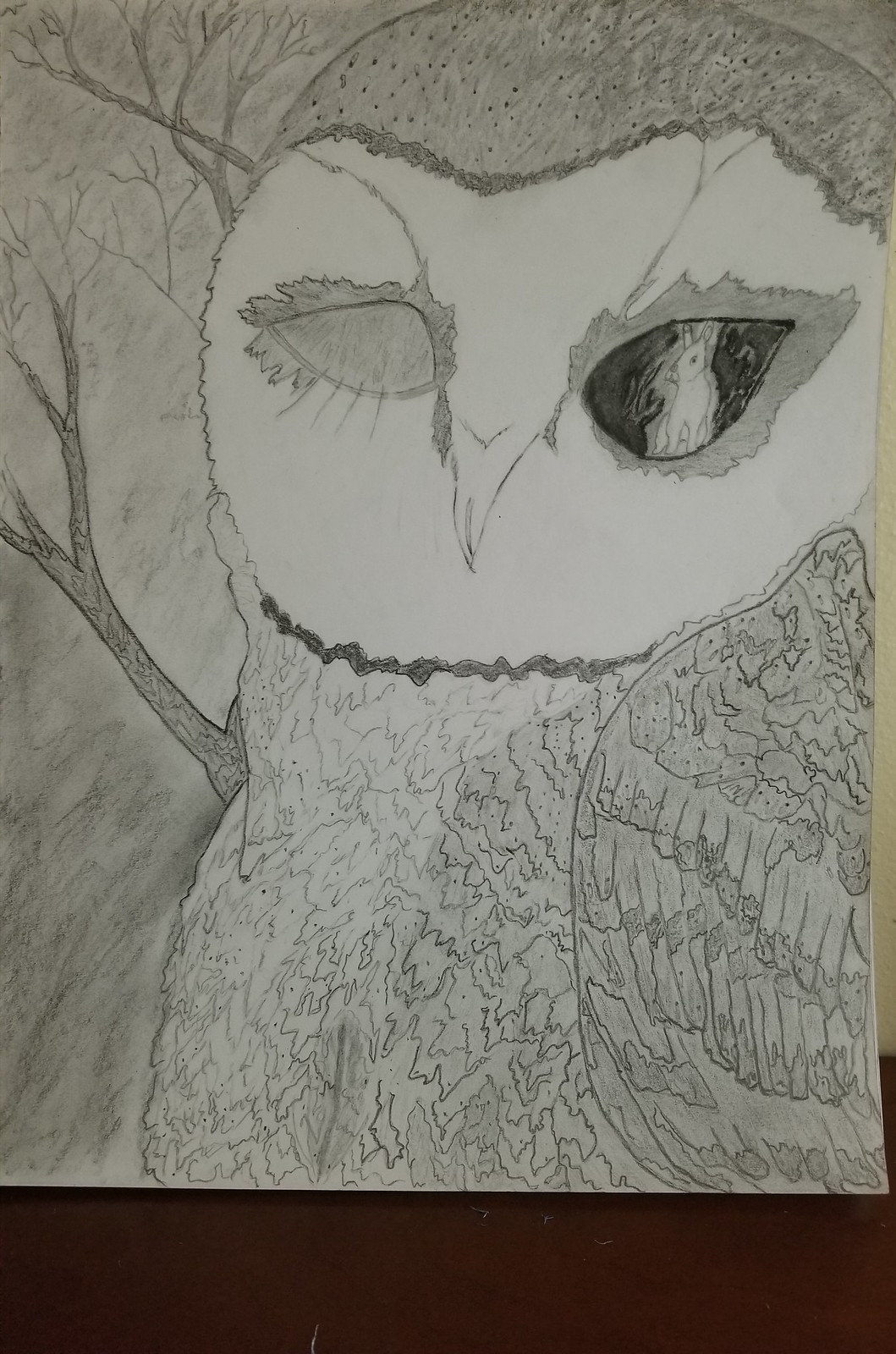This is a highly detailed pencil drawing of an owl, depicting its head and extending down to the middle of its chest. The owl is positioned facing left but its intense gaze is directed forward towards the viewer. Its eyes are almost teardrop-shaped; the left eye appears to be completely grayed out, perhaps closed or shaded, while from the right eye emanates a detailed reflection of a rabbit, suggesting the owl spotting its prey. 

The top of the owl's head features feathering with gray shadows interspersed with small black dots. It also has a slightly curved and shaded upper head above a distinctive white face. The bird's beak is triangular, and the chest feathers range in color from white on the left side to a more grayish hue on the right. Some feathers around the neck have a finger-like appearance, adding to the texture and depth of the image.

The background includes bare trees on the left side, enhancing the natural setting of the drawing. The overall ambiance of the image is monochromatic, done in shades of grey, suggesting it was drawn with pencil. This striking piece is completed on a white sheet of paper, which rests upon a dark surface, possibly a black or brown desk, emphasizing the illustration's details.